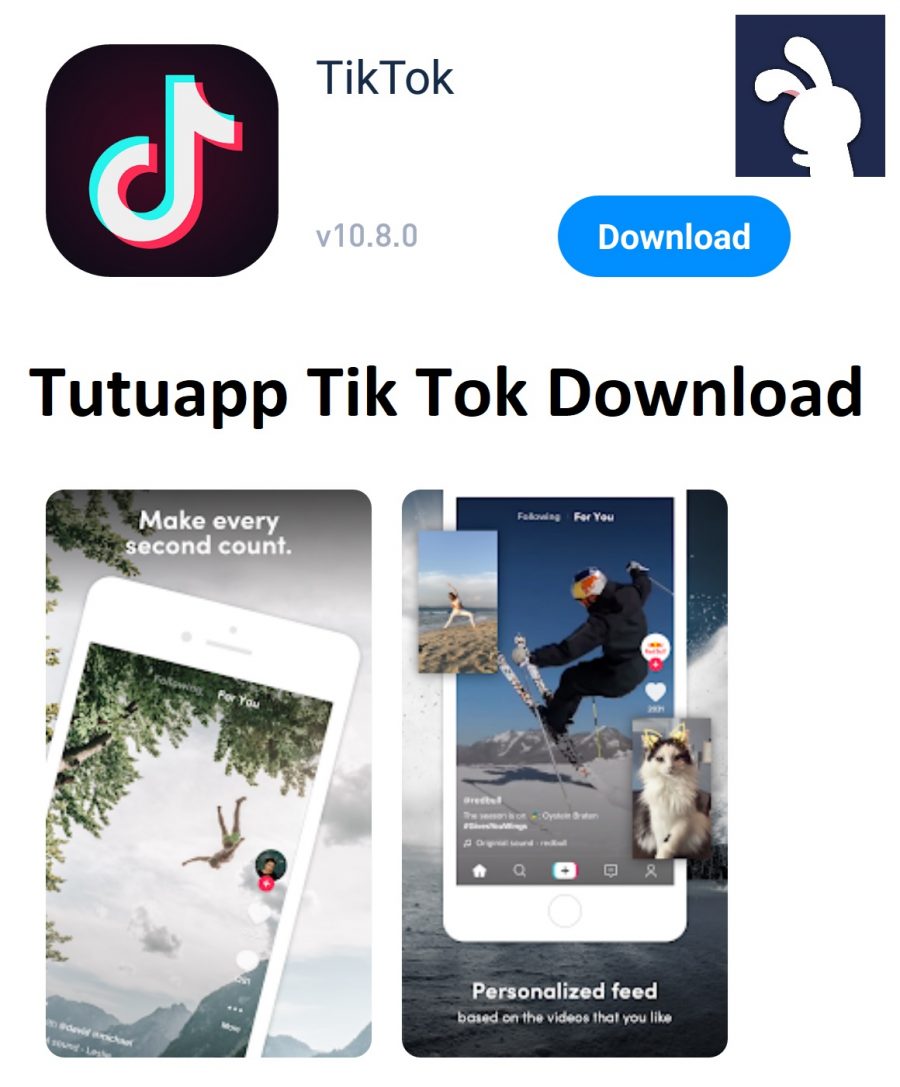This is a detailed screenshot from an app store for the TikTok application. In the top left corner of the screenshot, the TikTok logo is prominently displayed, directly followed by the word "TikTok" in dark navy blue, almost black text. Beneath this text, in a smaller and lighter gray font, is the version number "V10.8.0".

In the upper right section of the screenshot, there is a dark blue box containing a white silhouette of a bunny rabbit. Below this box, there is a rounded oval blue button with white text that reads "Download".

Occupying the middle section of the screenshot is a bold, black headline that states, "TutuApp TikTok Download." Directly underneath this heading are two side-by-side screenshots. The first screenshot shows a phone displaying an image of a person falling from a tree, accompanied by the caption "Make every second count." The second screenshot features a phone set against an ocean backdrop, with an image of a person skiing and the caption "Personalized feed based on the videos that you like."